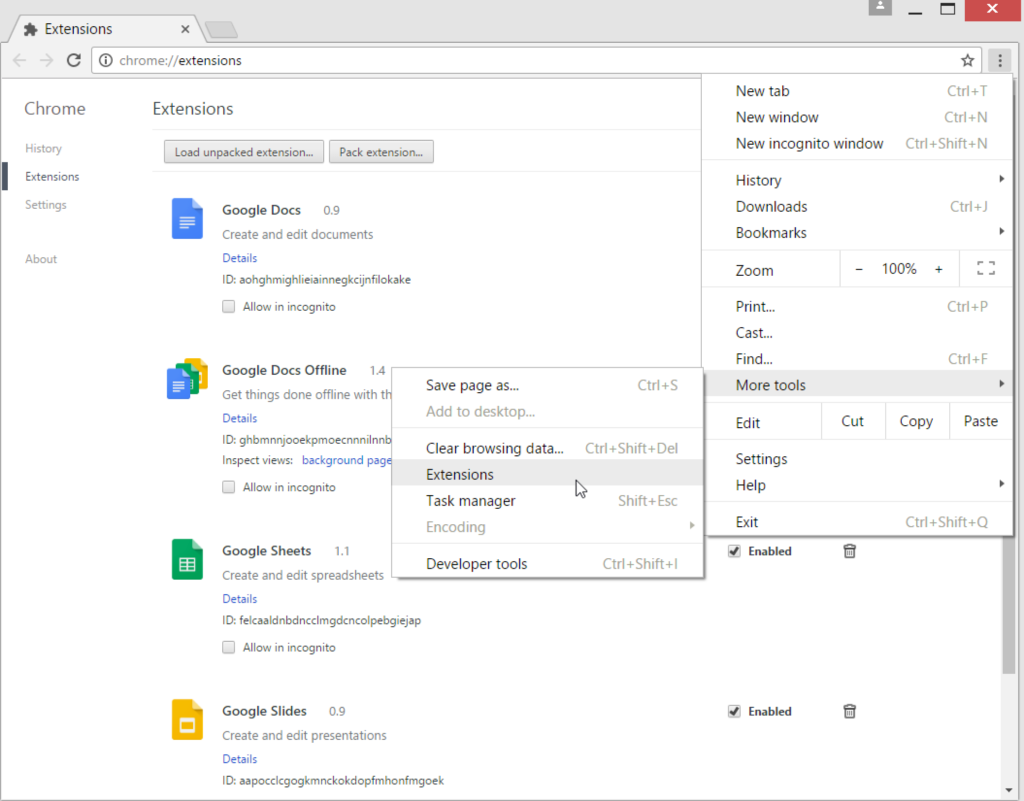This screenshot captures the Chrome web browser interface, specifically the 'Extensions' section. At the top, a grey banner runs across, with the active tab also grey and labeled 'Extensions.' Along the left side, a vertical menu displays several options: Chrome, History, Extensions, Settings, and About. The 'Extensions' option is bold, indicating it is currently selected.

On the right side of the browser, a series of drop-down menus are visible, showing that the user navigated through 'Settings,' selected 'More Tools,' and then chose 'Extensions.' The main content area features a detailed list of installed extensions. 

1. At the top of the list is 'Google Docs,' represented by a blue rectangle icon.
2. Below that is 'Google Docs Offline,' with a distinctive blue, green, and yellow document icon.
3. Next is 'Google Sheets,' identified by a green document icon with a spreadsheet symbol in the center.
4. The last visible extension is 'Google Slides,' which features a yellow document icon.

On the right side of each extension entry, there are checkboxes labeled 'Enabled', with two of them currently visible. Adjacent to these checkboxes are small trash bin icons, likely for removing the extensions.